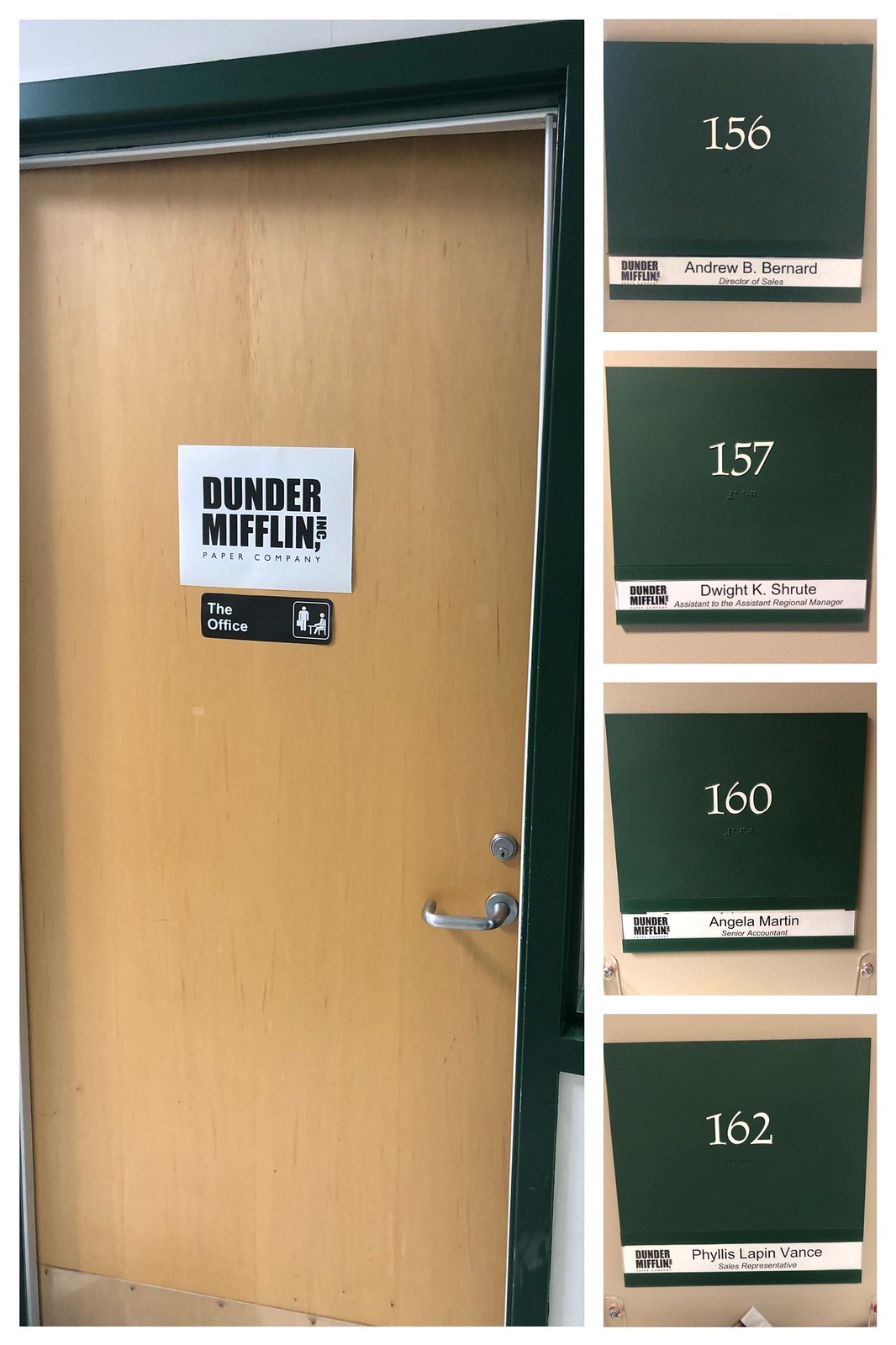The image depicts a wooden door with a black frame, positioned on the left side and partially open. Attached to the door is a white paper sign with black lettering that reads "Dunder Mifflin Inc. Paper Company." Below this is a small black placard with white text that says "The Office." The door features a metal kick panel at the bottom and has a handle, rather than a knob, for turning, with a lock positioned above it.

On the right side of the image, distinct from the door itself, are a series of green office nameplates displaying room numbers and names of individuals. The top nameplate reads "156" for Andrew B. Bernard, followed by "157" for Dwight K. Schrute, "160" for Angela Martin, and "162" for Phyllis Lapin Vance.